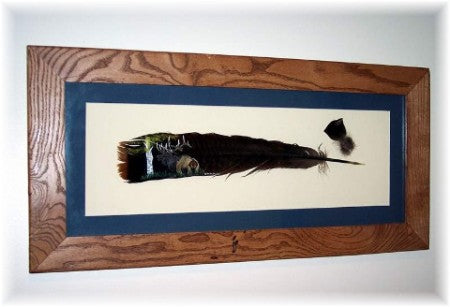The photograph showcases a unique piece of framed art. The frame itself is constructed from medium brown wood that could possibly be cherry, with a prominent wood grain that adds a textured, maze-like appearance. Inside the frame, there is a dark blue matting that provides a striking contrast to the off-white background. Centrally mounted is a large feather that appears to be a spectrum of colors, transitioning from black at the base to a greenish hue with a white stripe near the top, and then back to black with hints of auburn at the very tip. Intriguingly, the feather features an intricately painted image of an elk, meticulously detailed to highlight its rear quarters and antlers. Accompanying the primary feather are smaller pieces that might also be feathers or related plumage, though their details are obscure in the lower resolution image. This piece, potentially an art exhibit, combines natural elements with artistic expression, offering a visually compelling display suitable for home decor.